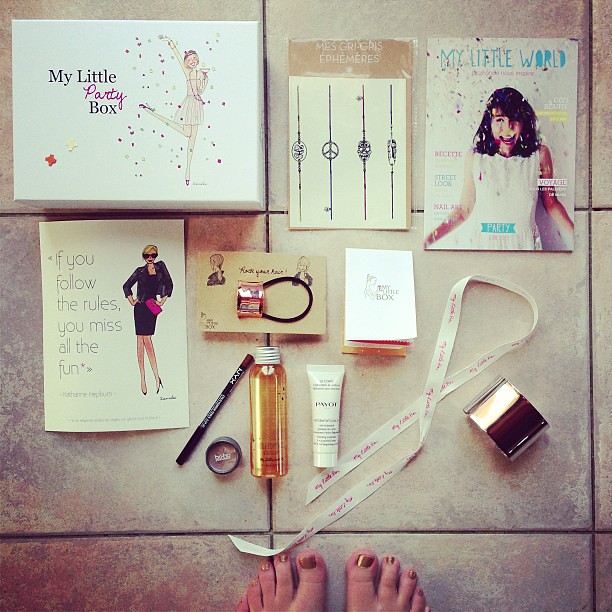The image depicts a collection of assorted items laid out on a white tile floor, organized in three rows. Centered at the bottom of the image are a woman's feet with gold nail polish. The top row features a decorated box, labeled "My Little Party Box," adorned with an illustration of a girl amidst glitter and confetti. To the right of the box lies another card depicting wristlets, labeled "My Little World," depicting a happy girl. The second row includes a card stating, "If you follow the rules, you miss all the fun," accompanied by a "girl boss" image. Positioned to the right of the card is a pink rose hair tie and another card. The third row showcases a range of beauty products: a beauty pencil, eyeshadow, a small bottle of orange liquid, a white beauty product tube, and a ribbon, followed by a photograph of feet with ten toes.